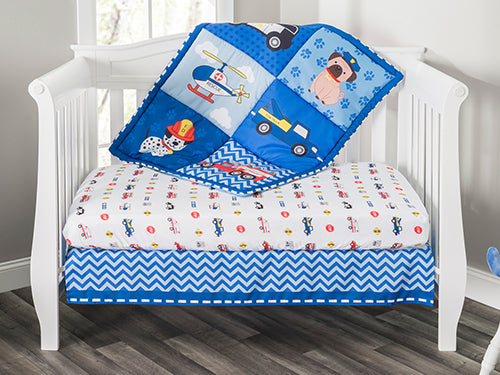The image depicts a cozy child's bedroom with light gray, rustic wood plank flooring and matching light gray-painted walls. The room features white molding along the floor and a window on the left wall with white trim, through which a glimpse of trees is visible outside. Central to the scene is a white crib placed in the corner of the room. The crib has a curved front and white slats along its sides and back, with one side of the crib open to display the inside details. The crib contains a mattress covered with a white sheet adorned with a variety of colorful small patterns, including cars, ambulances, and race cars. Beneath the mattress lies a fabric with a blue and white wavy or chevron pattern. Draped over the back of the crib is a blue blanket featuring six squares with different whimsical patterns, such as helicopters, pigs, dogs, trucks, police dogs, and firefighting dogs, all in a cartoony style.